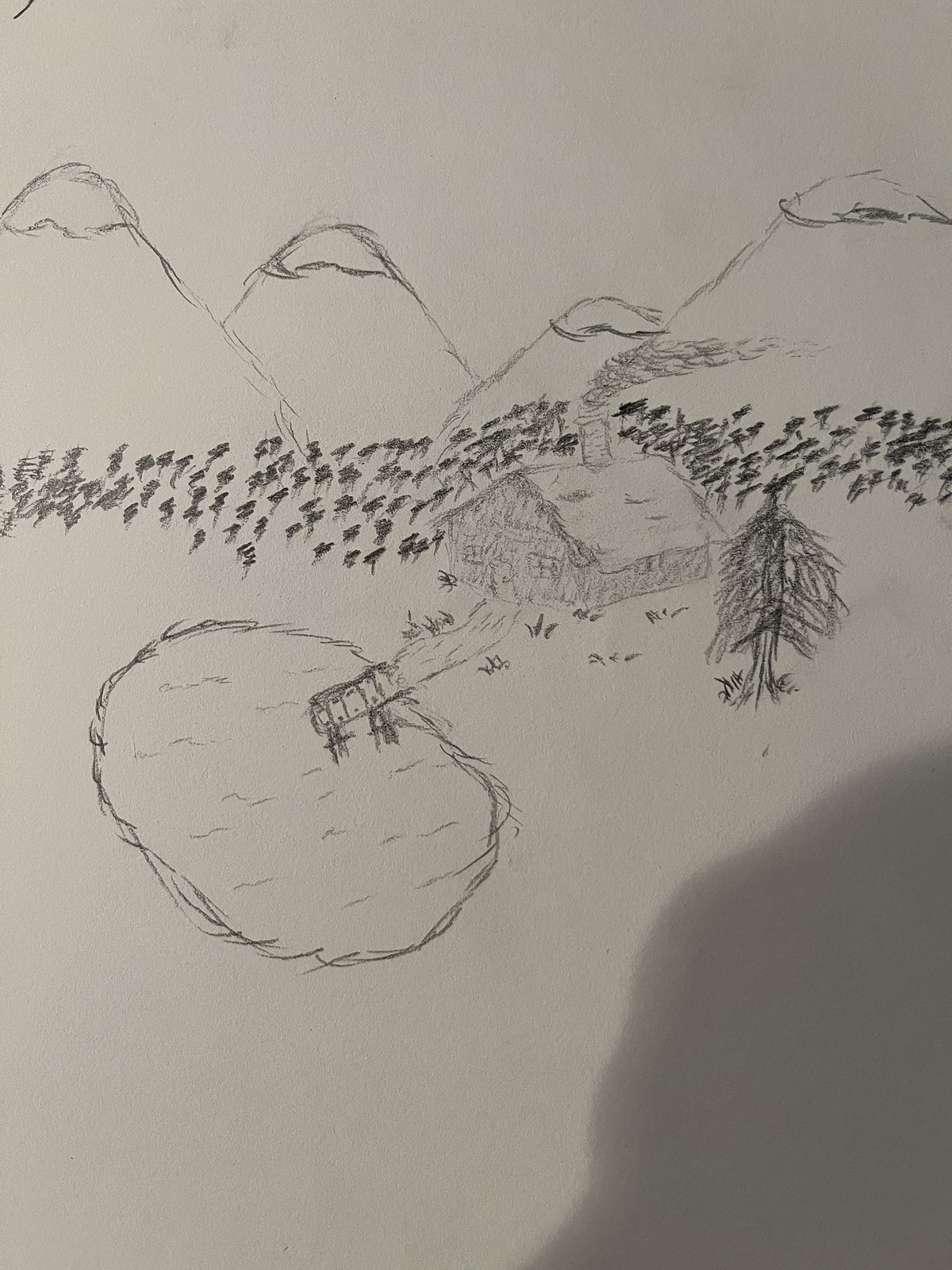This is a detailed pencil illustration on white paper depicting a tranquil lakeside scene with a shadow in the bottom right corner, likely from the person taking the photograph. Central to the drawing is a darkly shaded cabin featuring a slanted rooftop and a chimney emitting smoke, with two windows flanking a centered door. The cabin is nestled among small trees, with a more detailed tree with branches and leaves to its right. In the backdrop, large triangular mountains with snowcaps rise majestically, while beneath them, clusters of trees and forests provide a dense, natural setting. To the left of the cabin, a narrow walkway leads to the lakeside, where a small pier extends over the water. The lake itself is illustrated with wavy lines, indicating movement and small dashes to form its circular shape. Overall, the monochromatic sketch uses shades of gray to bring to life a serene nature scene with a remote cabin, reflecting both rustic charm and the artist's attention to natural elements.